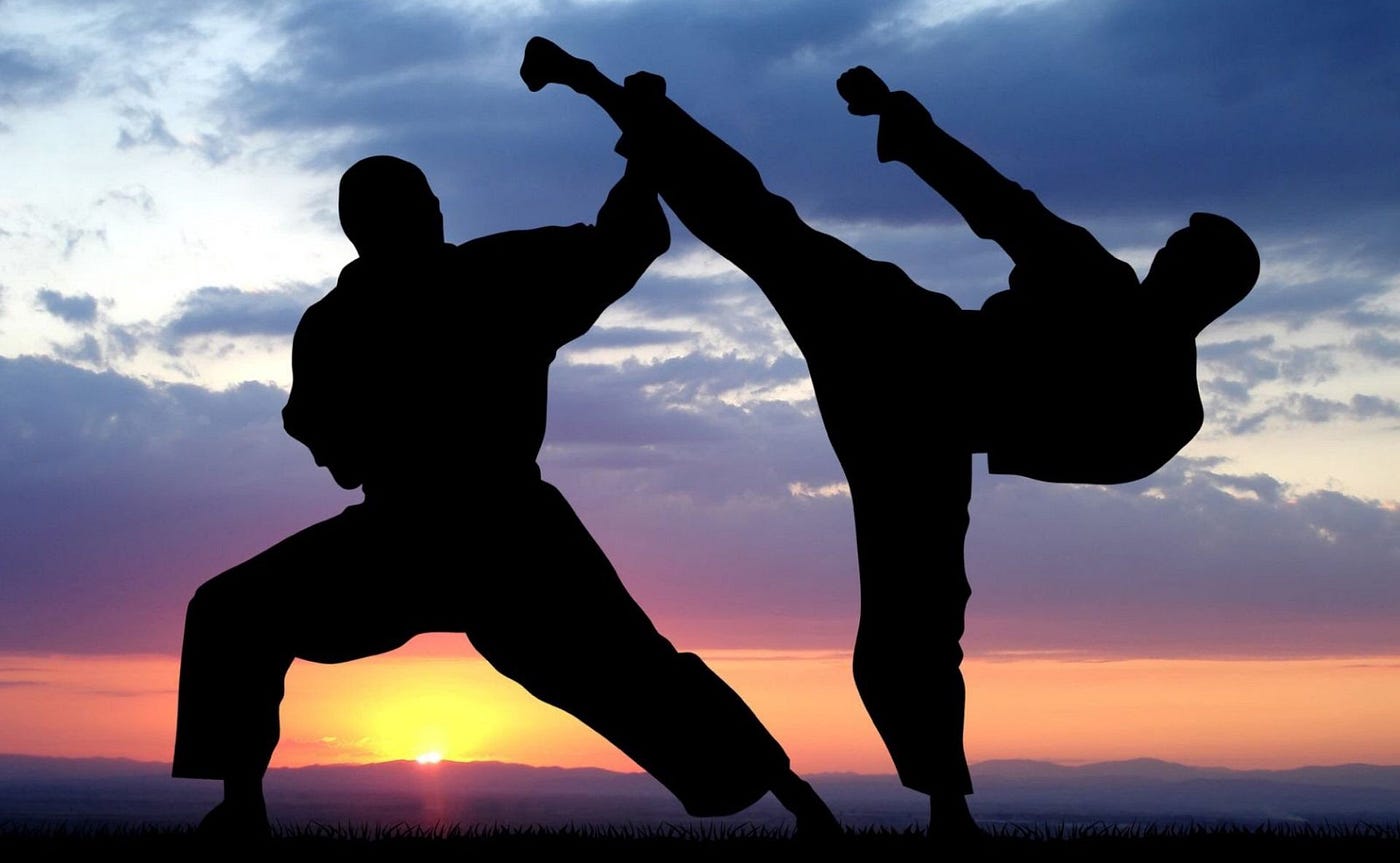The image portrays two men, silhouetted against a vibrant, multi-colored sky, practicing karate outdoors. The man on the right is executing a high kick with his right leg, while the man on the left is blocking the kick with his right arm. The backdrop, suggestive of either sunset or sunrise, features a stunning gradient of colors—ranging from deep blue at the top to bright orange and yellow near the horizon, accentuated by scattered clouds. The sun is prominently positioned near the bottom of the frame, casting a dramatic light that enhances the silhouettes of the men. Below the sky, a range of mountains stretches across the horizon, adding to the natural beauty captured in this clear and vividly illuminated photograph.